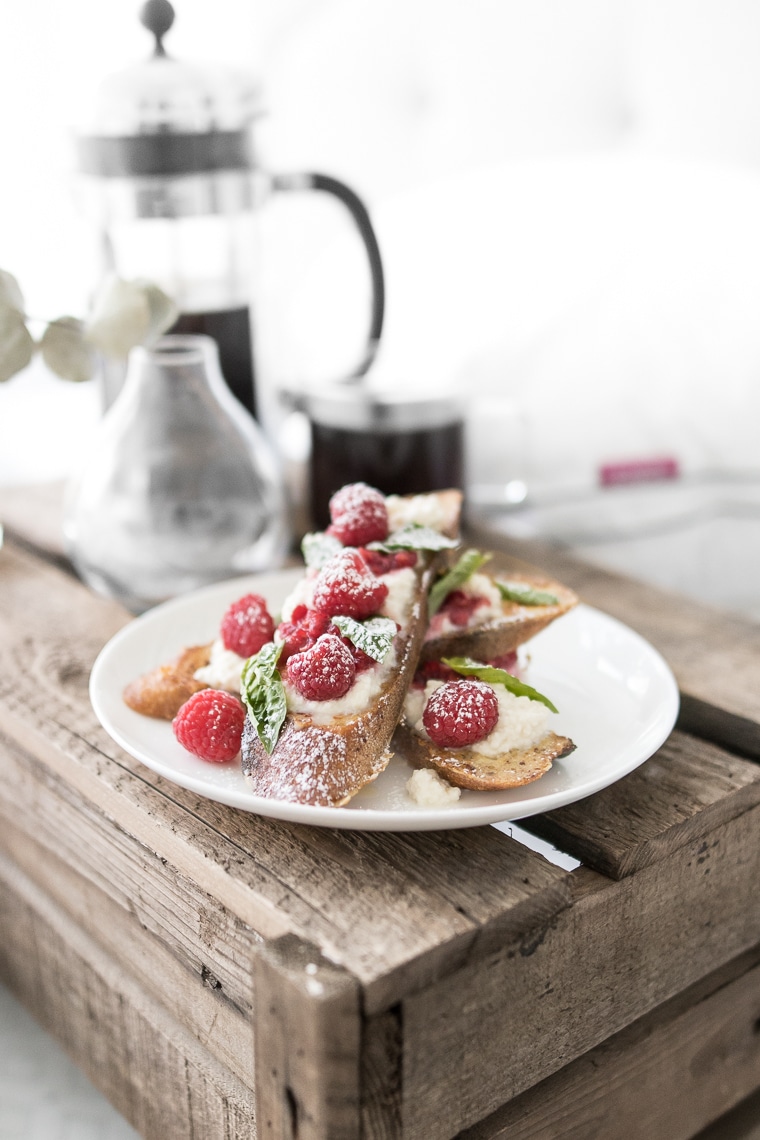The photograph is a professionally stylized and detailed composition featuring a delectable dessert. At the center of the image is a pristine white ceramic plate holding a slice of bread or cake, generously adorned with a creamy spread. On top of the spread lies an artistic arrangement of vibrant red raspberries, dusted with a light sprinkle of confectioners' sugar. Adding a burst of color, fresh green leaves, possibly basil or mint, are used as garnish. The plate rests on a rustic brown wooden crate, whose slats run both vertically and horizontally, providing a textured backdrop to the scene.

In the background, there is a meticulously arranged coffee set, including a French press full of rich, dark coffee and a glass cup already filled with the aromatic brew. To the left, a glass vase or possibly a candle holder, tapers elegantly at the top. An exquisite white flower peeks out from the upper left corner, adding a touch of natural elegance to the setting. The entire composition is framed against a clean white background, enhancing the prominence of the dessert plate and the harmonious balance of the colors and textures.